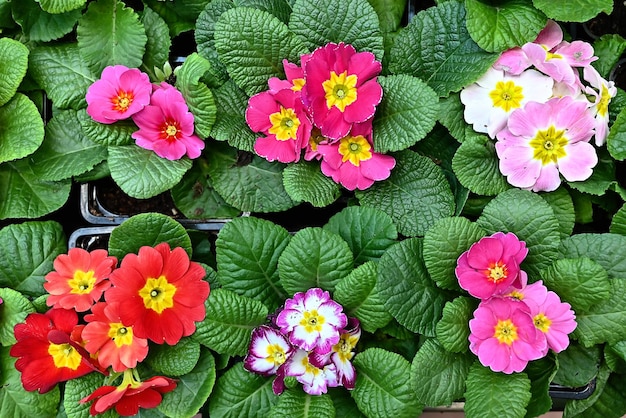This is a detailed, close-up aerial view of six vibrant primrose plants displayed in black plastic flats at a plant nursery. The rich green leaves surrounding the flowers add texture and depth to the composition. In the top row, from left to right, there are pink flowers with yellow centers, followed by another group of pink flowers featuring deeper pink hues. The rightmost plant in this row showcases lighter pink flowers along with a single white flower, all with yellow centers. The bottom row, from left to right, contains a cluster of red flowers with yellow centers, adjacent to purple flowers with white outer edges and yellow centers, and concluding with another group of pink flowers with yellow centers. The variety of colors, including fuchsia, red, white, and several shades of pink, creates a visually delightful spectrum. The leaves appear textured and lush, enhancing the overall beauty of the delicate blooms.